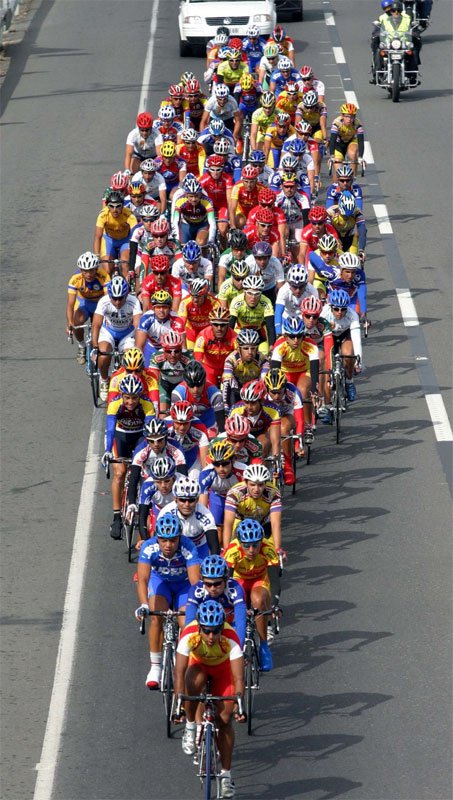The image depicts a dynamic scene of a biking event, likely part of a parade, showcasing a large group of cyclists meticulously arranged in a diamond formation on a two-lane road. The leader at the forefront is followed closely by rows of riders, all packed tightly together like sardines, creating a visually striking V-shape. They are all equipped with helmets featuring ventilation holes, and their colorful jerseys and helmets - in shades of yellow, red, blue, and white - add vibrant contrast to the setting. A distinct white line at the edge of the road and a brim mark the side, while in the background, a white car and a motorcycle can be seen following the cyclists, adding an element of motion and context to the event. All participants are facing towards the viewer, enhancing the immersive and engaging nature of the photograph.